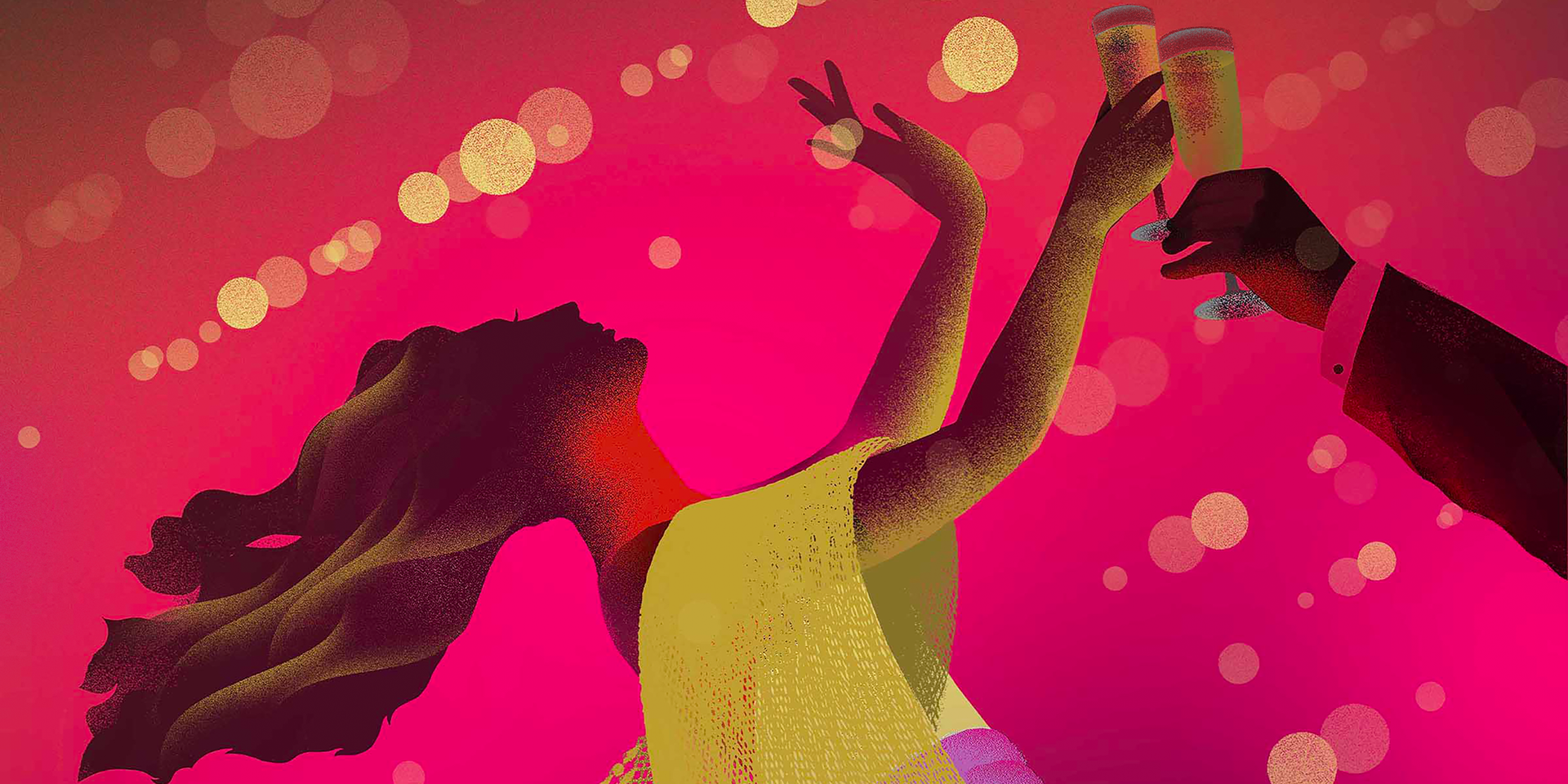The digital image showcases a pixelated, shadowy scene set against a bright pink background with circles and lines resembling reflections from bright lights, evoking a lively atmosphere, possibly a nightclub. At the center is a woman with flowing dark brown hair, caught mid-twirl, adding to the dynamic feel of the picture. She appears to be joyfully partying, holding a glass of champagne with her right hand raised. She wears a striking yellow dress or shawl, draped over one shoulder, featuring large, stylish sleeves. To the right, a man’s arm, clad in a suit with the shirt's cuff and button visible, extends into the frame, also holding a glass of champagne, suggesting a celebratory toast between the two.